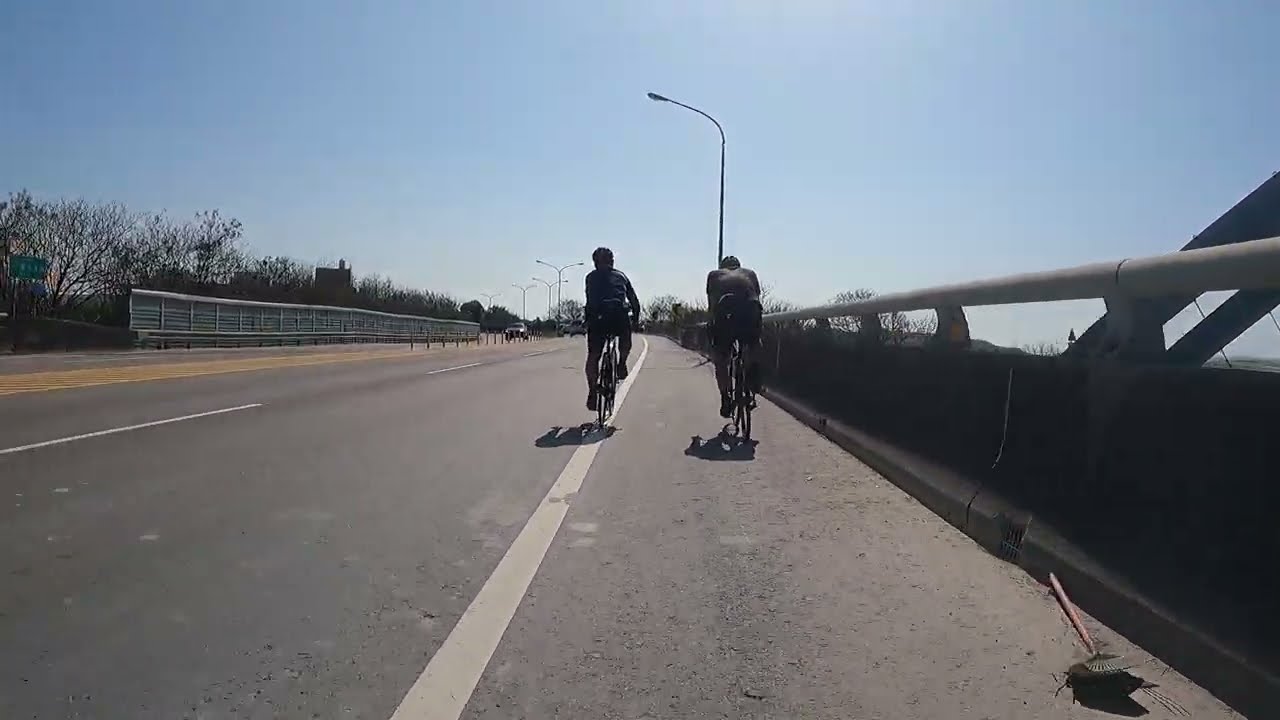In this detailed photograph, two bikers clad in black and gray attire and wearing helmets are viewed from behind as they ride side by side along the shoulder of a divided four-lane highway. Both their bicycles are also black. The highway, featuring a black asphalt road with a dotted white center line dividing lanes and a yellow separator for the directions of traffic, appears to be on a bridge or overpass, evident by the railings flanking the scene. The clear, sunny day with blue skies highlights the leafless winter trees in the distance. Streetlights and a street sign are visible ahead, while a lone car approaches in the oncoming traffic lane. A peculiar detail—a broom—lies abandoned on the roadside immediately to the right of the riders, adding an unexpected element to the otherwise orderly scene.